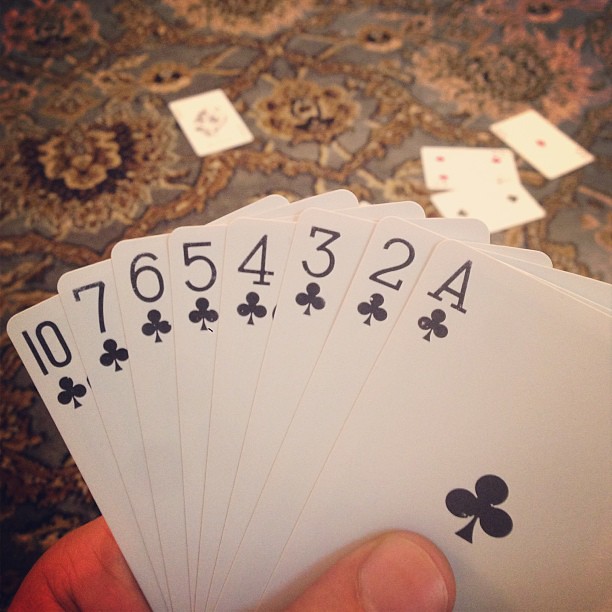A detailed photograph captures the moment as someone holds a hand of playing cards. The cards are simple and white, displaying a variety of clubs: an ace, two, three, four, five, six, seven, and ten, lined up from ace on the right to ten on the left, though they aren't in a straight sequence. The person's thumb and fingers are visible, pinching the cards and fanning them out from their perspective.

In the background, a blurred ornate pattern suggests an oriental rug with paisley prints and floral designs in shades of blue, gold, brown, and black, though it could also be a tablecloth. Scattered on this surface are additional playing cards—a partial spread that includes a diamond, a possible two of clubs, an ace of diamonds, a four of hearts or diamonds, and perhaps a joker. The game being played is unclear, but it evokes the feel of an intimate card game, possibly rummy. The intricate background and scattered cards add depth and context to the scene, emphasizing the close-up focus on the player's hand.